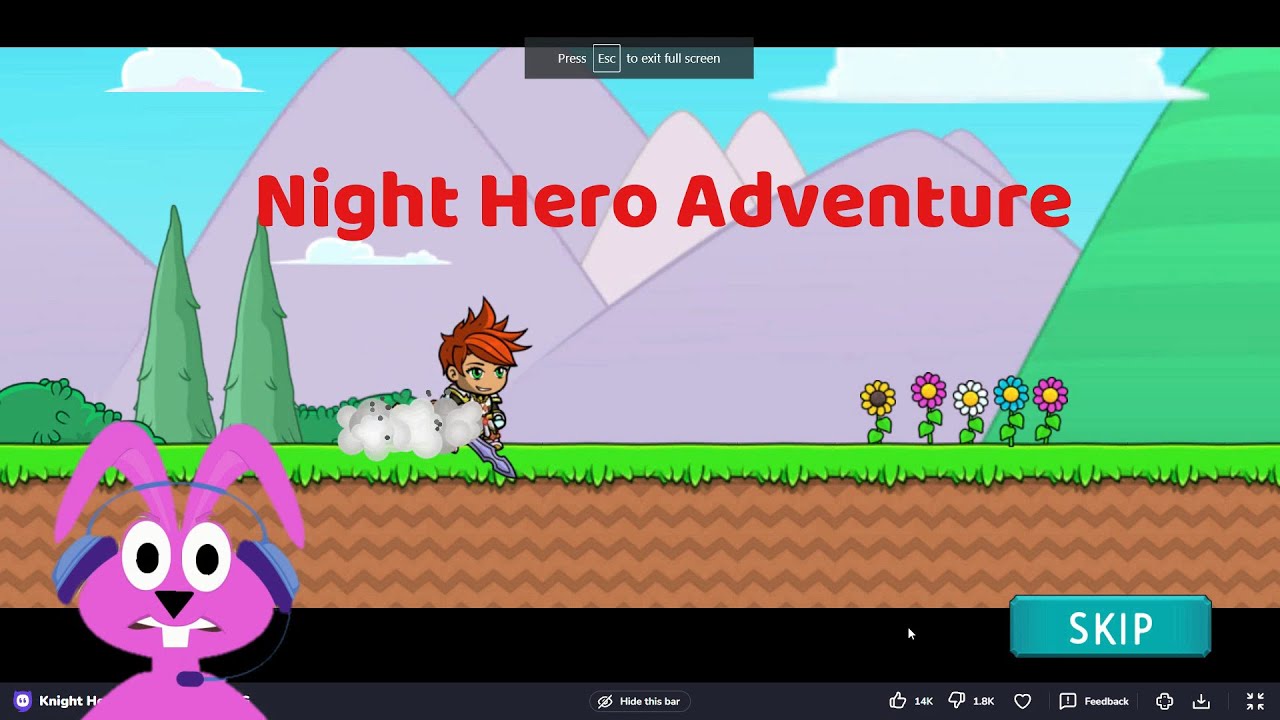The image is a rectangular screenshot from a video game titled "Knight Hero Adventure," written in red text across the screen. The scene showcases a cartoon avatar character with red, spiky hair, wielding a small sword, and walking along a grassy area adorned with flowers. The flowers are varied in color: two purple with yellow centers, a yellow one with a dark center, a white one with a yellow center, and a blue one with a yellow center. The background features a tranquil landscape of mountains, green hills, and trees under a blue sky with clouds. The grass area is depicted with an underlying brown dirt layer.

On the bottom left of the image, a purple bunny character appears to be engaging with the game, wearing blue and purple headphones with a microphone. A notable feature on the screen includes a rectangular blue "Skip" button in the bottom right. Additionally, the bottom of the image displays various interactive icons such as likes, dislikes, hearts, feedback, and save options, along with text indicating, "Press Escape to exit fullscreen."